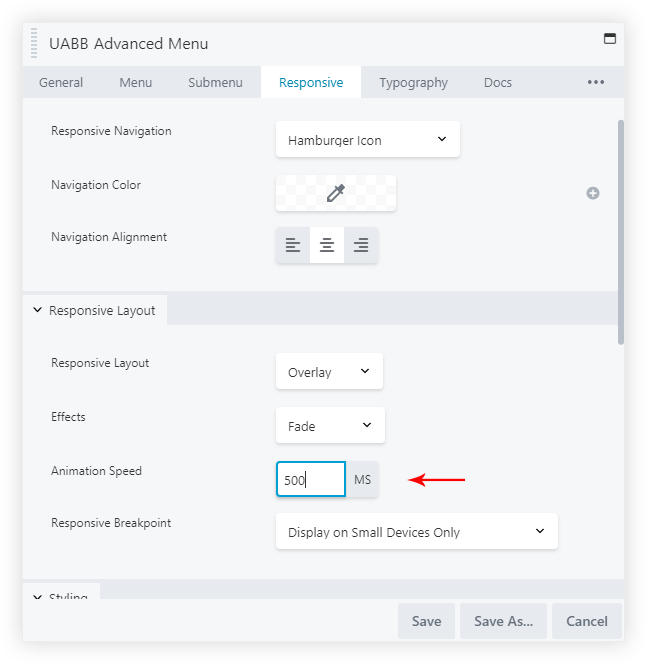Screenshot of a computer screen displaying the 'UABB Advanced Menu' interface, set against a gray background. At the top, the menu options are visible, including 'General', 'Submenu', 'Responsive' (highlighted in teal), 'Topography', and 'Docs'. Below this menu, a gray box outlines various settings under the 'Responsive' category. These settings include:

- 'Navigation' with a 'Hamburger Icon' option visible.
- 'Navigation Color' and 'Navigation Alignment', both showing no selected options.
- 'Responsive Layout' with several sub-options: 'Responsive Layout' again and 'Overlay', both with no selected options.
- 'Effects', which is set to 'Fade' with an animation speed of '500 ms'. This section is highlighted with a teal outline box and emphasized with a large red arrow pointing to it.
- 'Responsive Breakpoint', set to 'Display on small devices only'.

At the bottom of the gray box are three buttons: 'Save', 'Save As', and 'Cancel', completing the interface view.